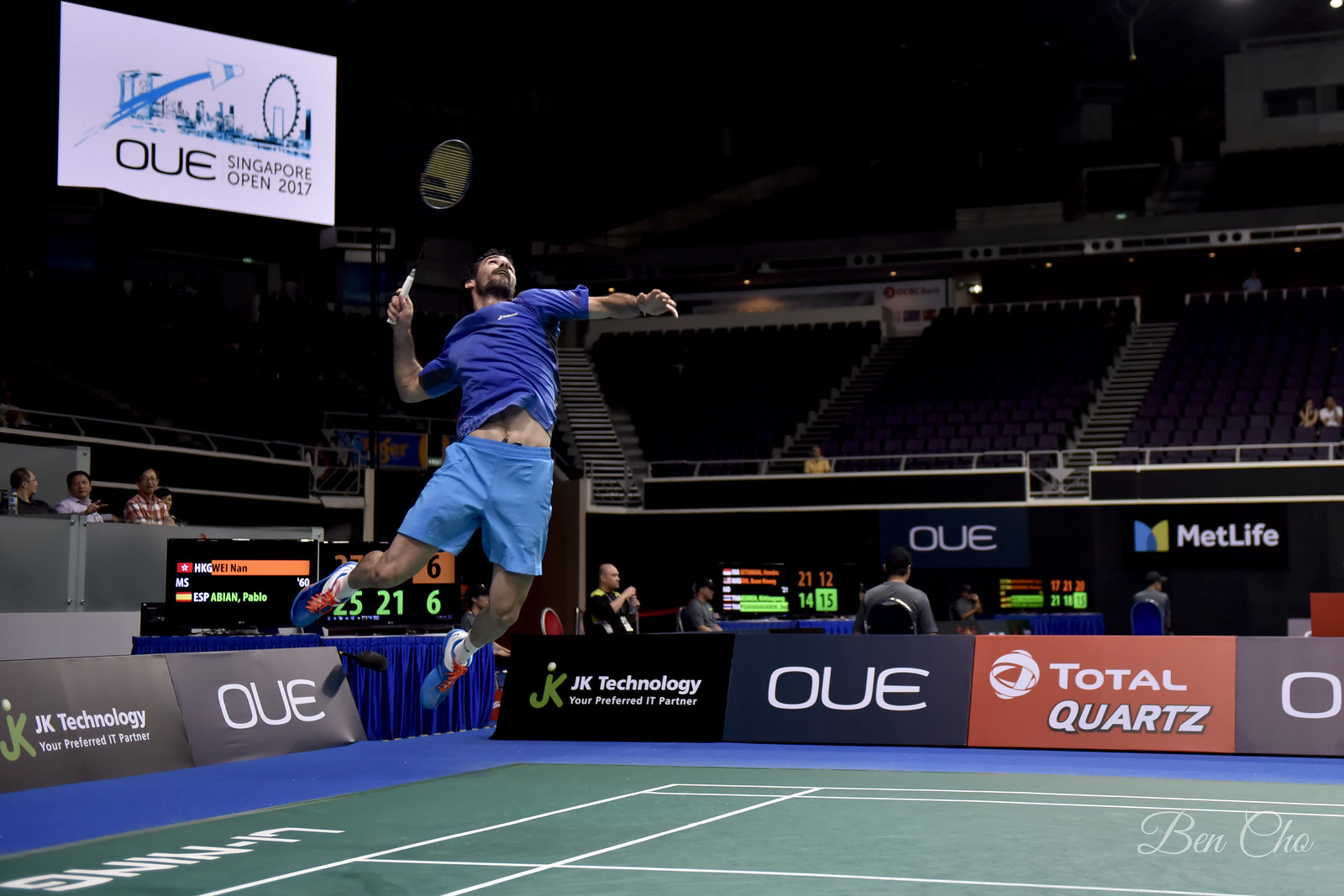This is a detailed photograph depicting a badminton player at the Singapore Open 2017, captured midair as he prepares to strike the shuttlecock. The player is sporting a dark blue shirt, light blue shorts, and blue sneakers with orange laces. His right arm is cocked with a racket in hand, while his left arm extends horizontally, parallel to the court. The vibrant badminton court features a green in-bounds area bordered by blue out-of-bounds sections and white lines. The stadium, though large, is mostly empty with only a few spectators scattered about. Numerous banners and advertisements, including those for JK Technology and Total Courts, adorn the surroundings, and a banner bearing "OUE Singapore Open 2017" can be seen hanging from the top left of the frame. In the bottom right corner, there's a credit to the photographer, Ben Cho.